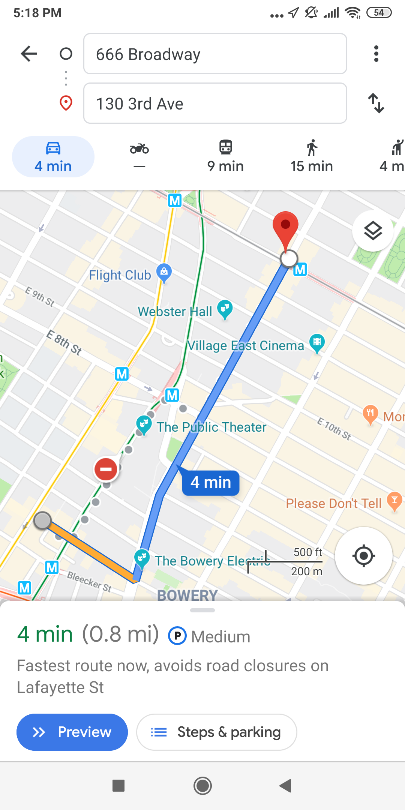The screenshot displays a Google Maps route with detailed navigation information. At the top, there is a left-pointing arrow accompanied by a text box indicating the destination, which is entered as "666 Broadway" with an open circle next to it on the left. Adjacent to this, three vertical dots are visible, followed by a red pin symbol. Further to the right, another text box shows "133rd Ave" with an up and down arrow next to it, signifying the option to reverse the route.

Below the destination section, various transportation symbols are displayed: a car icon with "4 min," a motorcycle icon with a dash, a train icon with "9 min," a pedestrian icon with "15 min," and another pedestrian icon resembling a person hailing a taxi, marked "4 min."

The map itself illustrates a straightforward route: travel straight down one road and continue straight on another. Below this visual route, it reads "4 min (0.8 miles)" followed by a "P" in a blue circle with the label "medium." A note below this states: "Fastest route now. Avoids road closures on Lafayette Street."

At the bottom of the screenshot, a blue button with two arrows pointing to the right is labeled "Preview," and a white button labeled "Steps in Parking" is to the right, with some blue lines next to it. Finally, a compass symbol and a white circle button for readjusting the map are located in the bottom right-hand corner.